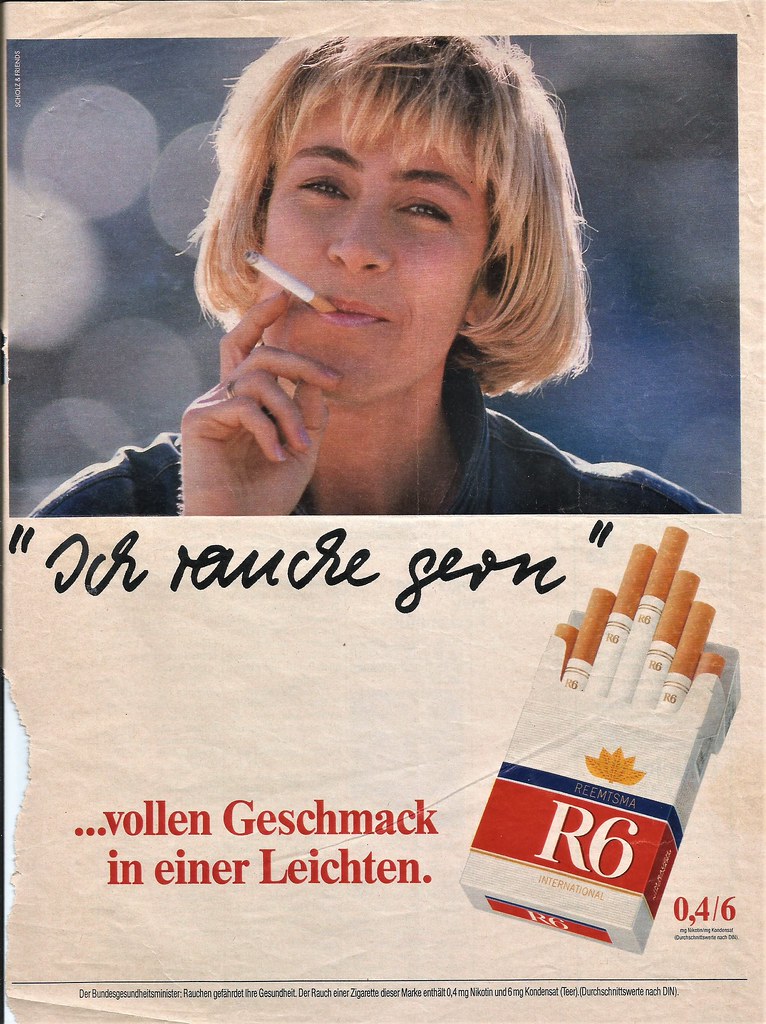The image showcases a vintage cigarette advertisement that appears to have been ripped from an old magazine or newspaper, with visible tearing along the left edge. The advertisement is predominantly in German, featuring bold, cursive text that is difficult to decipher, alongside the phrase "Vollen Geschmack in Einer Leuchten." The centerpiece of the ad is a vibrant and happy blonde woman with a bob haircut, hazel eyes, and pink frosty lipstick, typical of the 1980s style. She is smiling with a cigarette in her mouth, and her right hand with pink fingernail polish is raised near her face. To the right of her image is an open pack of R6 cigarettes, arranged in a triangular or pyramid shape. The cigarette pack is white, accented with red and blue, and adorned with a gold leaf logo.